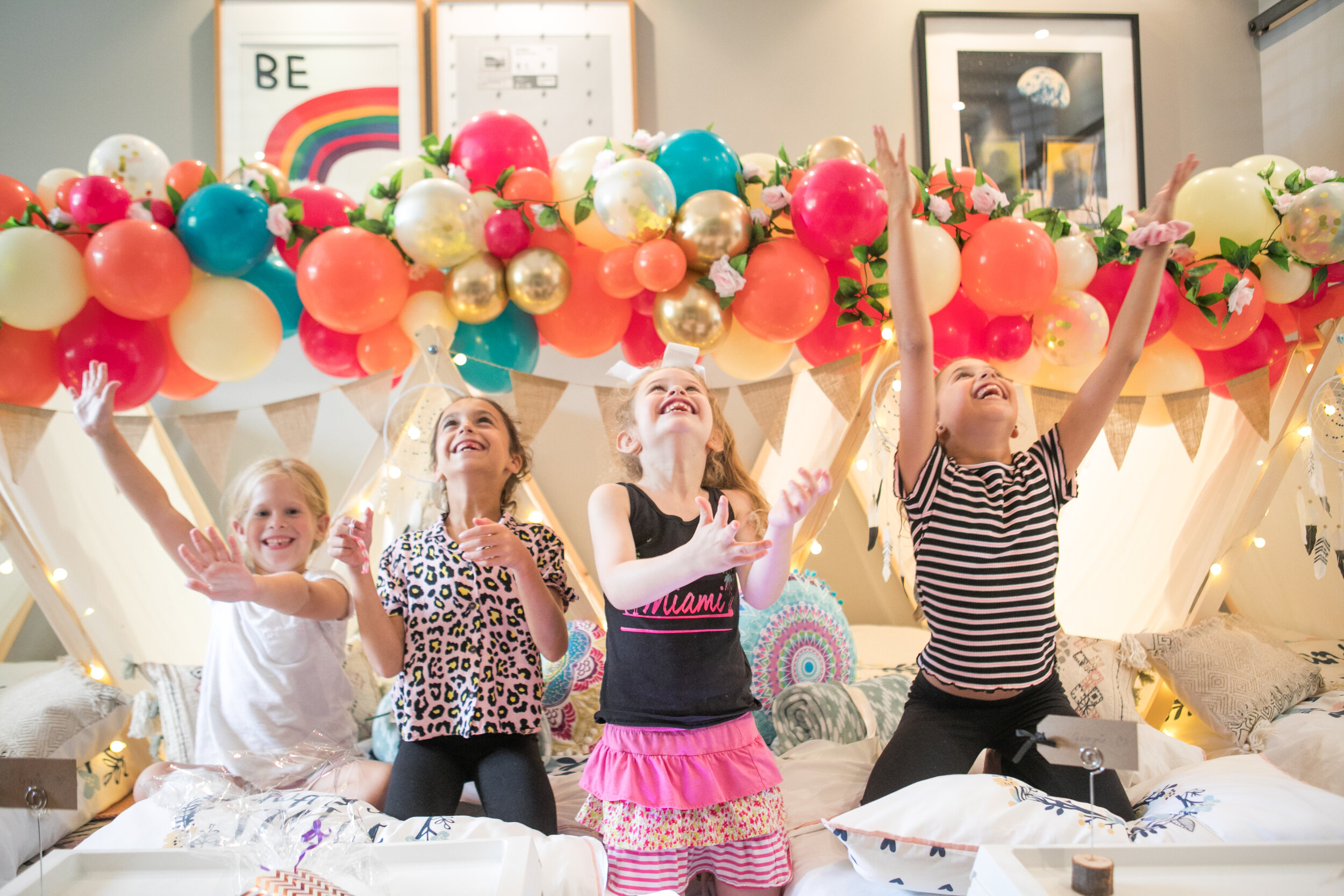The photograph captures a lively scene of four young children in the midst of a joyful celebration, likely a birthday party. The children are positioned at the forefront, all energetically waving their hands in the air and laughing. They are sitting on what appears to be a bed or couch, with various cushions in front of them and a decorative backdrop filled with colorful balloons in shades of yellow, orange, green, blue, and red hanging above.

From left to right: the first child is a girl dressed in a white shirt, who is the only one looking directly at the camera. Next to her is another girl in a leopard print shirt and dark gray or black pants, also gazing upward. The third child is a girl with a black shirt that has "Miami" printed on it and a pink skirt, her blonde hair visible as she looks towards the ceiling. The final child on the right is a boy, distinguished by his black and white striped shirt with black pants, equally engaged with the festivities.

Behind the children, the background includes a gray wall adorned with framed artwork. One of the frames features the letter "B," another showcases a rainbow, a third has black dots arranged in rows on a white canvas, and the last depicts the Earth from space. The combination of the children's animated expressions, the vivid balloons, and the artistic backdrop creates a vibrant and celebratory atmosphere in the photograph.